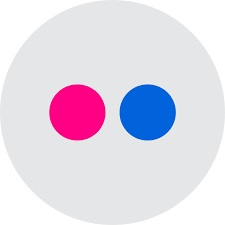This image features a large, solid light gray circle serving as the background. Within the light gray circle, there are two smaller circles: one is a vibrant, solid pink and the other is a deep, solid blue. These two smaller circles are positioned side by side and evenly spaced within the larger gray circle. The composition of the image presents a visually balanced arrangement of one large light gray circle containing one bright pink circle and one vibrant blue circle.